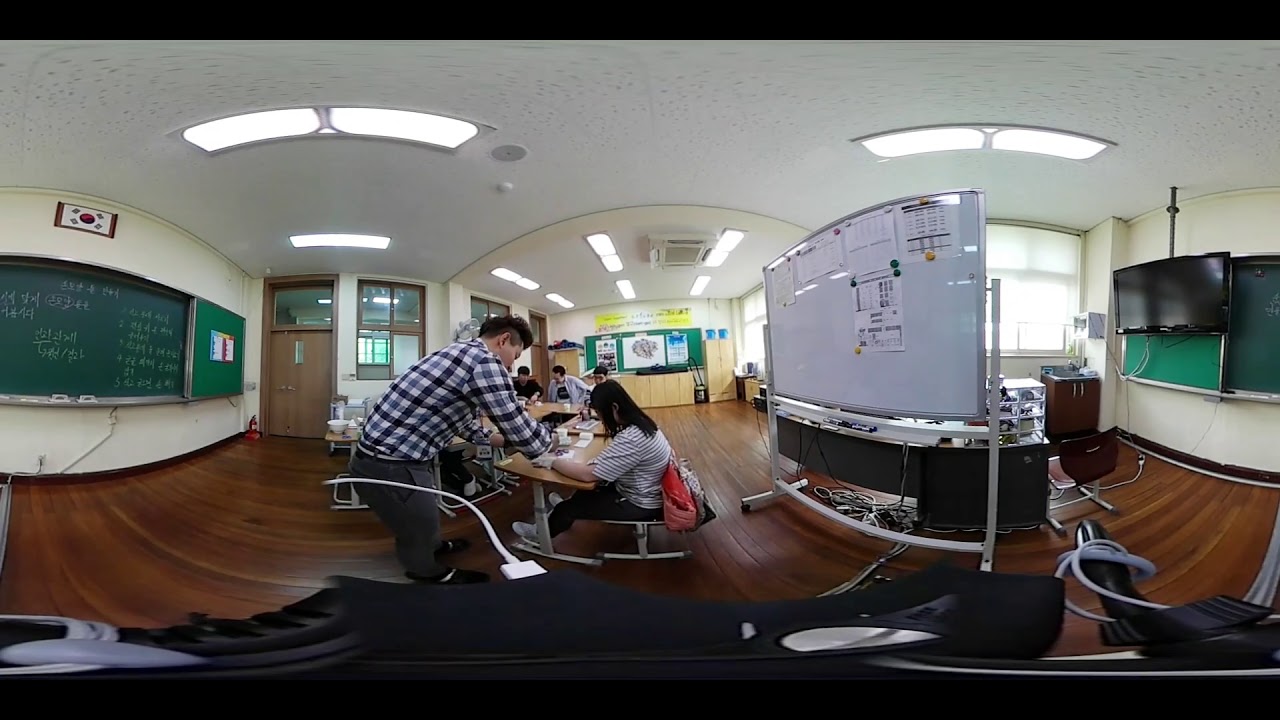This is a detailed photograph of a spacious classroom, captured from a wide-angle perspective. The room features dark hardwood floors and white ceilings, which are brightly lit. The walls are painted yellow, adding a warm ambiance. 

Several students are seated at individual tables, engaged in study, while one student stands out, wearing a black, white, and slightly blue checkered long-sleeved shirt paired with gray long pants. Directly in front of him sits a girl with short black hair resting just past her shoulders. She is wearing a black and white striped shirt, long black pants, and gray tennis shoes; a backpack is draped over the back of her chair, suggesting a comfortable and studious atmosphere.

On the left side of the room, there is a green chalkboard adorned with white chalk marks of Korean text, above which hangs a South Korean flag. Another green chalkboard can be seen in the back right, partially obscured by a rolling whiteboard and a TV. The whiteboard and additional chalkboards suggest a rich array of instructional materials. Audio-visual equipment is also present, enhancing the learning environment. The photograph illustrates a dynamic and multicultural educational setting that emphasizes active learning.